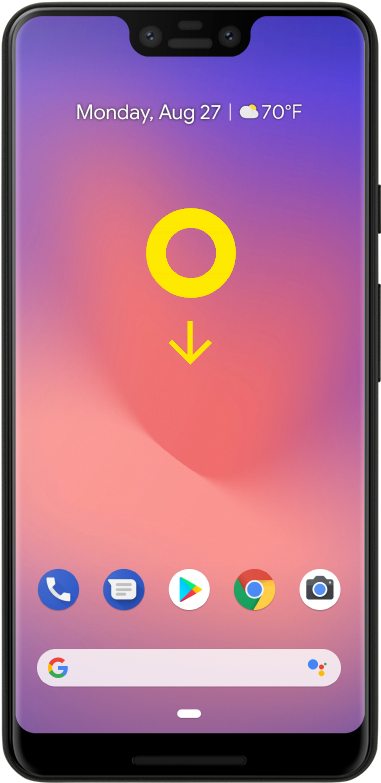The image is a vertically-oriented photograph of a smartphone. The phone features a black rim, with a lighter gray strip that’s particularly noticeable at the top and subtly extends down the sides. Near the bottom, the rim darkens to a deeper black, crossed by a thin gray line. 

The smartphone showcases dual cameras positioned on the top left corner, set within a small black insert that descends slightly into the phone. The two cameras are represented by two black circles, accompanied by two gray lines—one shorter above and a slightly longer one below.

The phone's screen displays an ombre background, transitioning from shades of purple at the top to hues of pink, peach, and salmon in the middle, and returning to a purple-pink gradient at the bottom. 

At the top of the screen, white text reads "Monday, August 27th" with a small vertical line beneath it. Next to the date is a cloud icon followed by "70 degrees Fahrenheit." A yellow circle with a downward-pointing yellow arrow appears below this information. 

Iconography along the bottom of the screen includes a phone symbol, a triangle, the Chrome browser icon, a camera icon, and a 'G' for Google. Below these icons sits a search bar, completing the detailed information depicted on the smartphone's display.